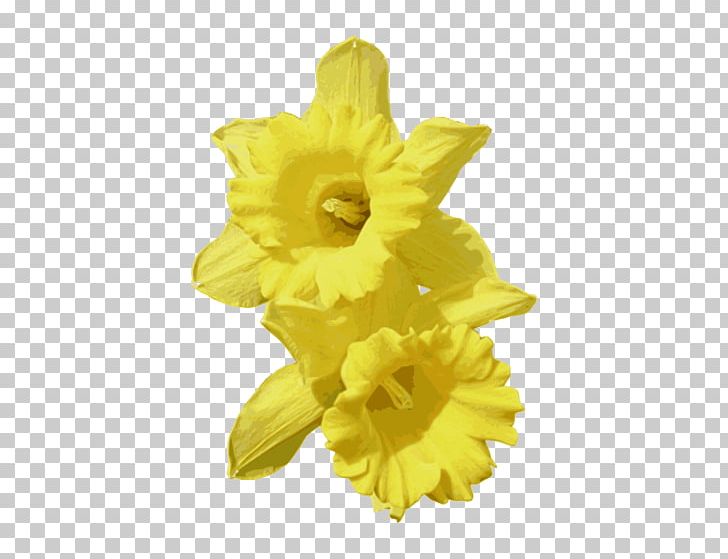The image depicts a highly realistic and meticulously detailed portrayal of two yellow daffodil blossoms set against a gray and white checkerboard background comprised of small squares. The daffodils, which occupy much of the central area, exhibit a palette of yellow hues that range from soft pastel shades with a touch of orange to deep, shadowed tones approaching black in the throats of the flowers. These blossoms have prominent trumpet-shaped coronas with intricate ruffled edges, and behind each are six delicate, horizontal petals. The entire composition is well-balanced, presenting a harmonious blend of vibrant floral elements and a muted geometric backdrop, enhancing the striking beauty of the daffodils.